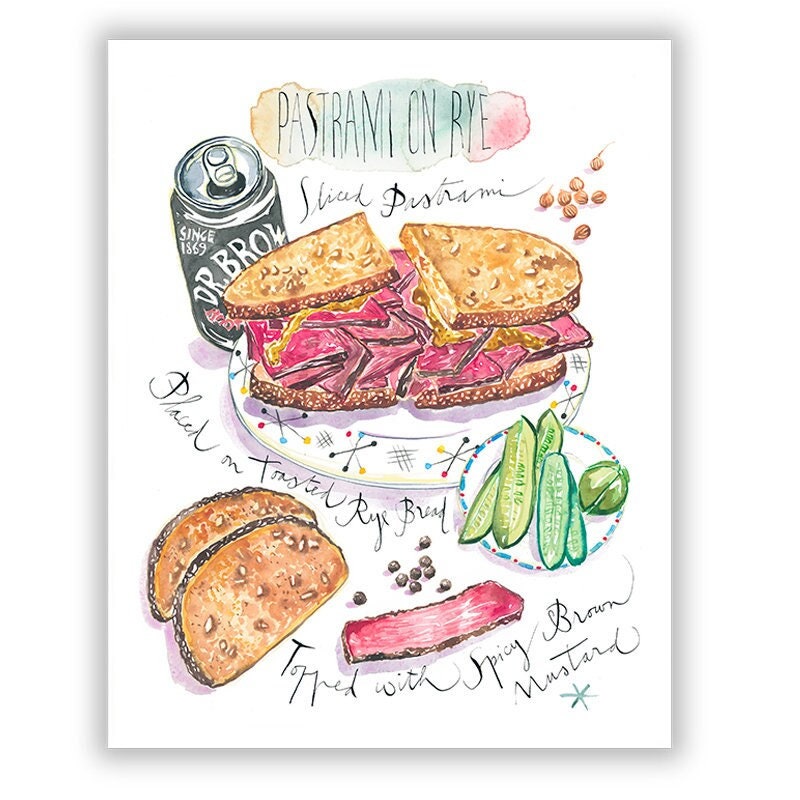This detailed watercolor drawing depicts a greeting card with a delectable lunch composition. At the top, in all capital black letters against a golden, blue, and reddish cloud background, the text reads "PASTRAMI ON RYE". Below, it states “sliced pastrami placed on toasted rye bread topped with spicy brown mustard,” accurately describing the featured pastrami sandwich. The sandwich, set on a plate adorned with a multicolored jacks border, is complemented by sliced green pickles on a side plate to its right. To the left of the sandwich, there's a can of Dr. Brown's soda, bearing a black background and the inscription “since 1869”. The artistic rendering captures the essence of a classic Jewish deli meal, presenting a visually appetizing scene on a white background.